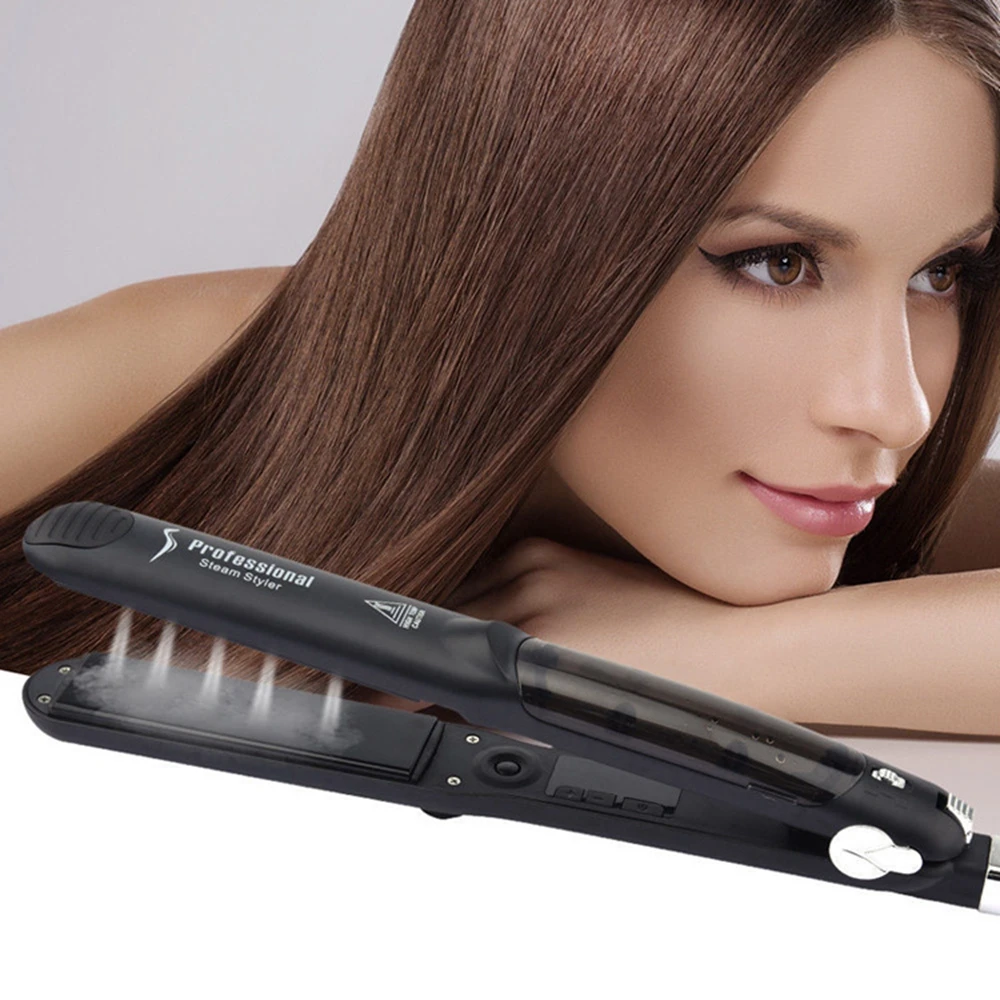The image is an advertisement for a women's styling brush, specifically a professional steam styler. The overall design of the styler is sleek and black, with "Professional Steam Styler" written in bold white text along the top. The steam styler features five jets of steam emitting from the area between its two prongs, adding to its modern and high-tech appeal. A whitish chrome hinge enhances its sophisticated design. 

In the background, there is a fair-skinned woman, resting her chin on the back of her left hand and gazing thoughtfully to her left. Her straight brown hair cascades gracefully over her right shoulder, with a few strands framing the left side of her face. She has captivating brown eyes and softly pink lips, adding a touch of elegance to the scene. The backdrop is a clean, whitish color, which accentuates the professional and polished look of the steam styler.